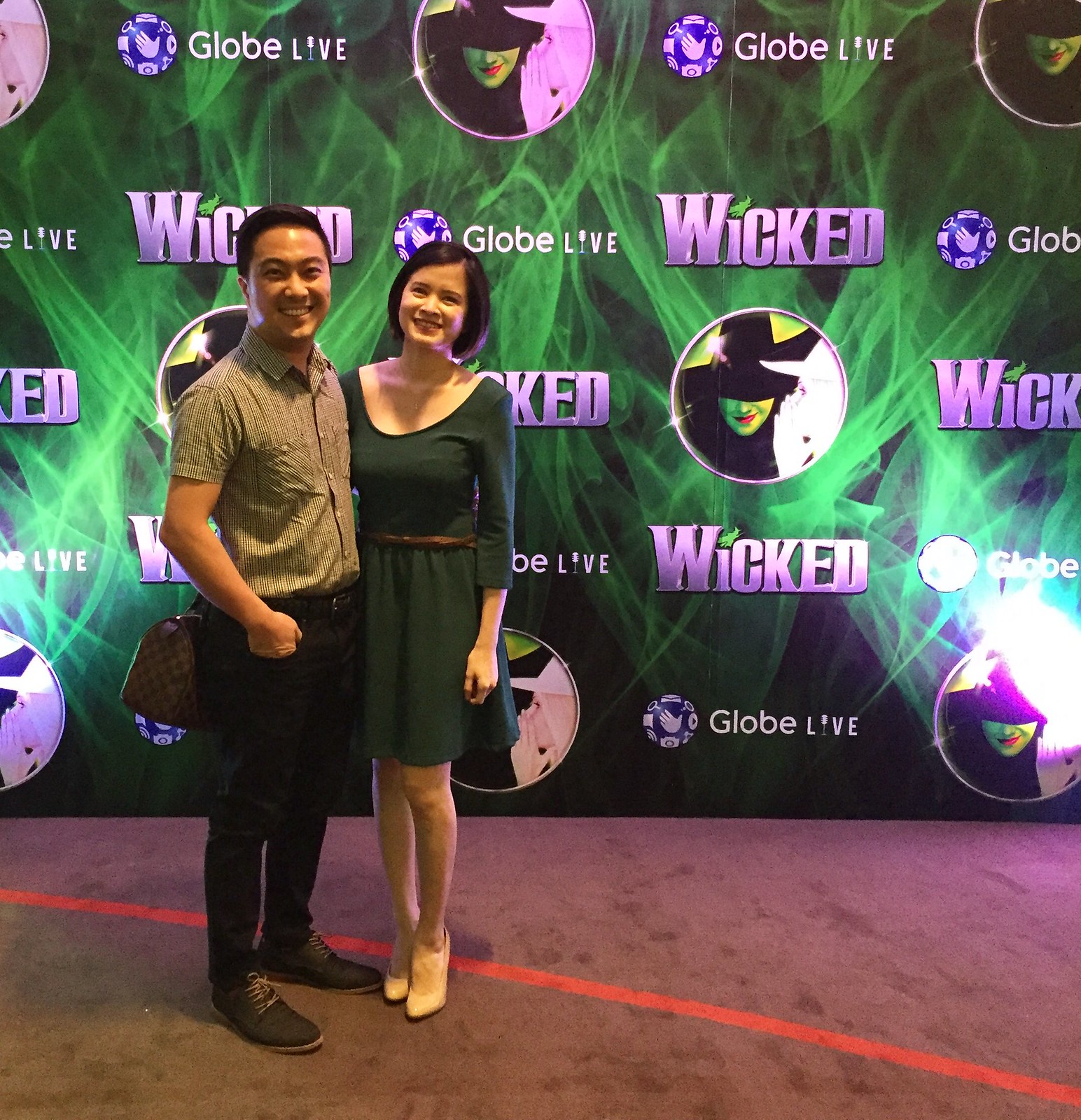In this image, the setting appears to be indoors, likely at an event. It features a carpeted floor as the ground surface. The background prominently displays a premiere panel for the musical "Wicked," with the logo "Globe Live" and a striking image of two witches— one with green skin in black attire and one in white, whispering into the other's ear. Off to the left side of the image stands a couple, slightly centered. The man, dressed in brown shoes, black pants, and a gray shirt, is smiling with his hands in his pockets. Beside him, a woman in a green dress and white high heels has her arm on his shoulder, also smiling at the camera. The color palette of the scene includes brown, red, black, gray, green, tan, purple, and white, enhancing the vibrant and cheerful atmosphere of the event captured in this photograph.